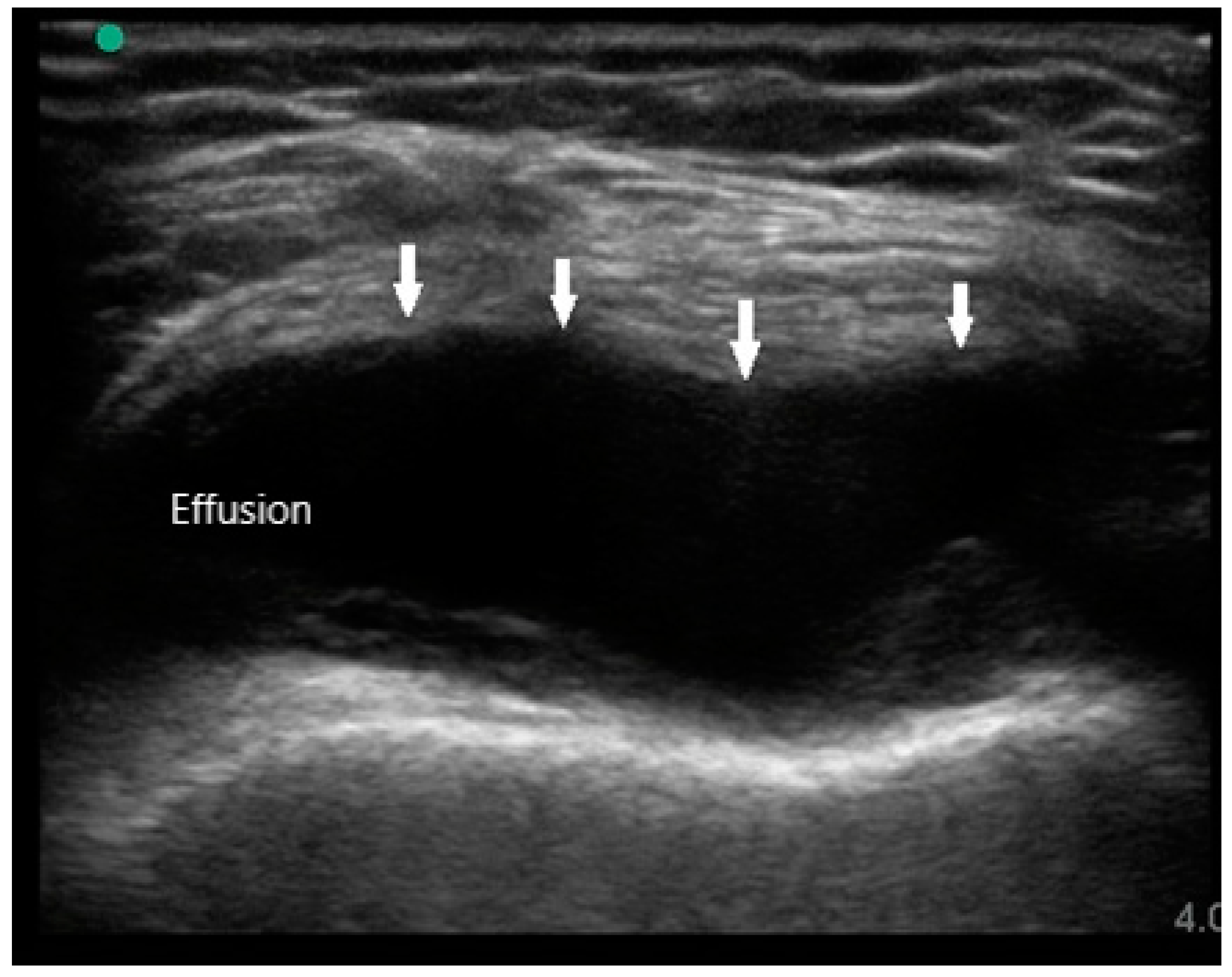The image is a black-and-white medical scan, likely an ultrasound or x-ray, showing a detailed view inside a human body. The setting is stylus medical imagery. The scan is almost square, with a slight landscape orientation, featuring thin black borders. At the center of the image, there is a dark, hollow section, resembling a river in a canyon, flanked by light gray, wavy, horizontal lines that form thicker bands at the top and the bottom. In this central dark area, the word "effusion" is written in a small white font. There are four white arrows pointing downwards towards this hollow section. A green circular dot is located in the top left corner of the image. Additionally, the number "4.0" appears in white at both the bottom left and bottom right corners, enhancing the detailed medical context of the photograph.